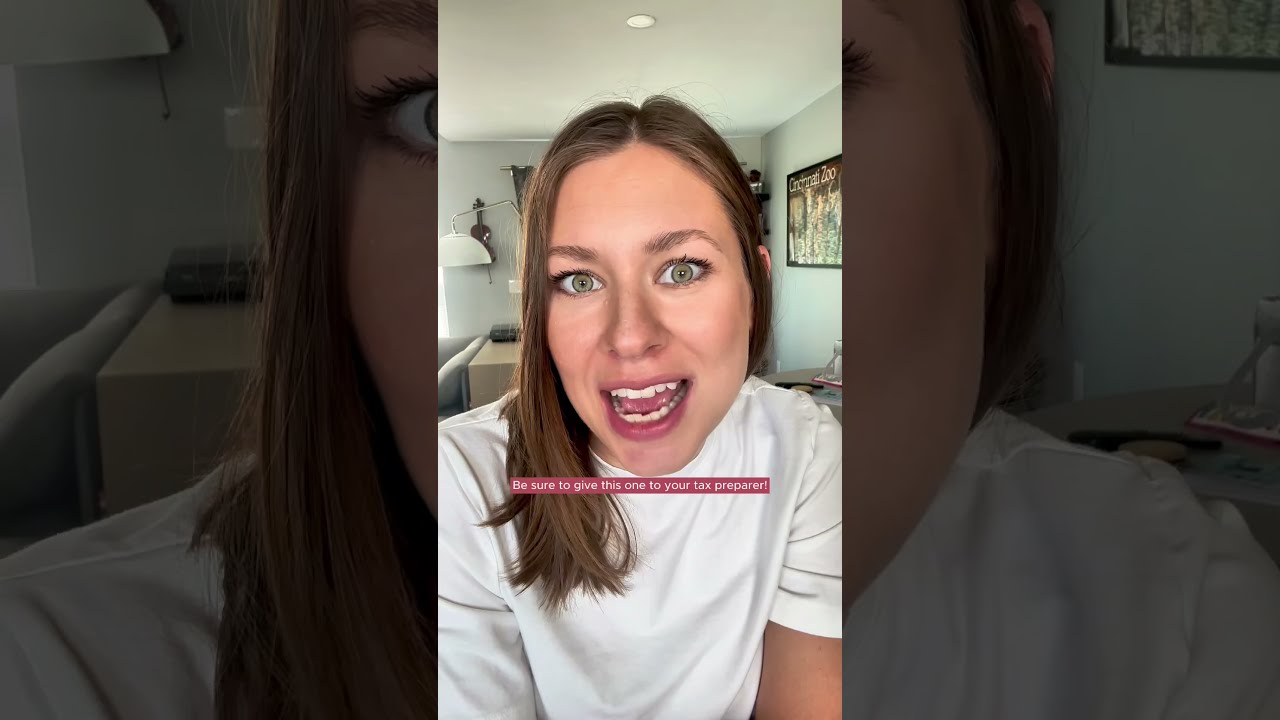The image captures a vertical photo, divided into three distinct sections. The two outer sections, shaded more darkly, feature a close-up of a woman's face split into left and right halves. The middle section, brighter and centered, reveals the full face of a woman in her 20s or 30s, with expressive green eyes and long brown hair, one side pulled back while the other side cascades down past her shoulder. She is clad in a white t-shirt and appears to be mid-speech, her mouth partially open, eyes wide, and teeth visible. 

She is situated in a home environment, likely a living room, illuminated by a white ceiling with recessed lighting. Behind her is a wall adorned with a piece of artwork and a visible lamp. To her side, additional home elements such as a gray couch with a gray pillow, a brown stand, and a corner of a chair can be discerned. The detailed background confirms the setting as a cozy, well-decorated room. Central to the image, just below her chin, is a small pink bar featuring a critical message in white text: "Be sure to give this one to your tax preparer!"